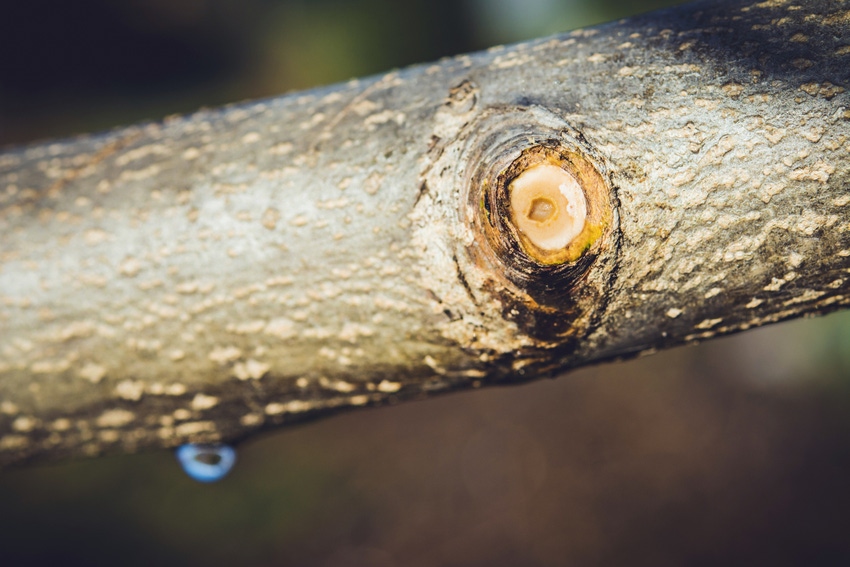The photograph is a detailed, zoomed-in, landscape-style macro shot of a tree branch, highlighting a recently pruned area where a twig or smaller branch was removed. The branch, approximately the size of a man's forearm, has a gray, textured bark with lighter, tan-colored ridges and a distinct cut revealing an exposed, whitish interior. The pruned spot is visibly leaking sap, forming a droplet that hangs noticeably at the bottom. There is also a greenish hue around the pruned area, possibly indicating the beginnings of moss. A noticeable blue segment, potentially a bug or water droplet, adds an unusual element to the scene. The background, out of focus due to the camera's aperture settings, consists of blurred greenery suggesting the presence of other trees and a clear, sunny day with light and shadow play evident on the branch.